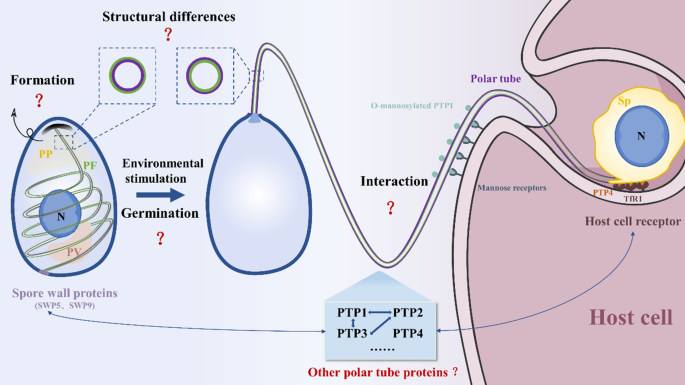The image is a scientific diagram with a light blue background, showcasing processes likely related to biology. At the top left, in black text, it says "structural differences." Below this, there are two small blue dotted boxes containing circles colored blue and green. Underneath these boxes are two larger light blue oval shapes. The left oval, labeled "formation," contains a swirling white line and a blue circle marked with an "N" inside it, surrounded by the annotations "PP" in yellow, "PF" in green, and "PY" in light pink, all collectively labeled as "spore wall proteins." Next to this oval, the phrase "environmental stimulation" is written with a blue arrow pointing right towards the next section labeled "germination," with a red mark under it.

The right half of the diagram features a pink area labeled "host cell." There's a tube connecting the left and right sides of the image, indicating interaction between these sections. Within the pink area, there's another oval shape, shaded yellow, containing a blue circle marked "N." This section is labeled with "polar tube" and "host cell receptor," indicating various structural and functional components of the host cell interaction. The diagram combines detailed annotations and color-coded processes to illustrate the differences and interactions in the biological processes depicted.